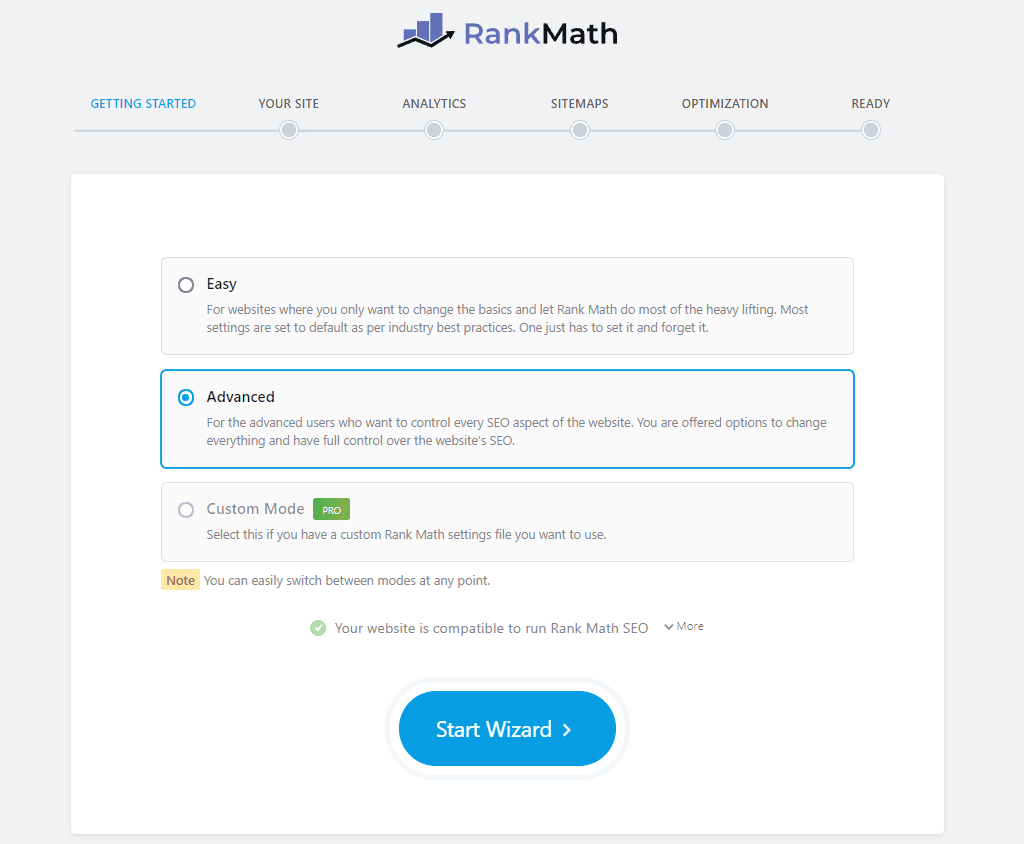The screenshot showcases a light gray website interface. Centrally positioned at the top is a blue bar graph icon featuring a small black arrow at its base. Adjacent to the icon, the word "Rank" appears in blue font, followed by "Math" in black. Directly below, a horizontal gray line separates the header from subsequent sections.

Above the gray line, the phrase "Getting Started" stands out in blue. To the right, categories such as "Your Site," "Analytics," "Sitemaps," and "Optimization Ready" are listed, each marked by a small gray circle beneath them. 

Further down, a white square panel occupies the main section of the screenshot. At the panel's top, a gray rectangle houses a small black circle labeled "Easy." The adjacent text describes this setting, emphasizing that it is ideal for users who prefer minimal adjustments, allowing Rank Math to handle most SEO tasks by default according to industry best practices.

Below this section, highlighted within a blue circle, the text "Advanced" is visible. This mode caters to users seeking comprehensive control over every SEO element of their website. The "Advanced" setting is currently selected.

At the bottom of the panel, "Custom Mode" is grayed out, indicating it is not active. A small red rectangle labeled "Pro" in white text is also present, signifying premium features or content.